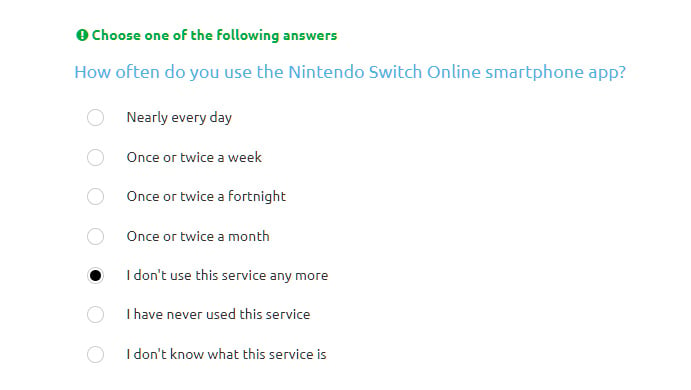The image has a white background and features a green circle with a white lowercase "i" at the top, possibly indicating an information icon. Next to the circle, in green text, it reads: "Choose one of the following answers." Below this, in light blue text, it poses the question: "How often do you use the Nintendo Switch online smartphone app?" There are several response options listed in black text, each separated by a blank line:

1. "Nearly every day."
2. "Once or twice a week."
3. "Once or twice a fortnight."
4. "Once or twice a month."
5. "I don't use this service anymore."

To the left of the line containing "I don't use this service anymore," there is a bold black circle indicating a selection. Following this option, the potential responses continue:

6. "I have never used this service."
7. "I don't know what this service is."

The lower portion of the image remains blank with no further text or elements.